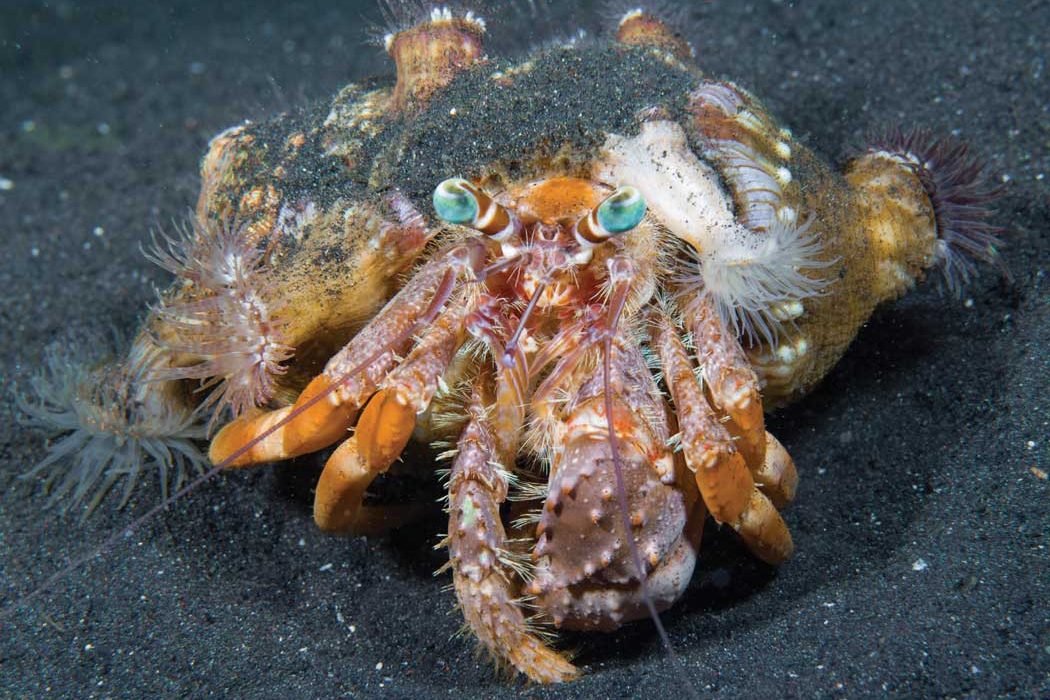This close-up photograph captures a fascinating sea creature half-burrowed in dark gray or black fine sand, speckled with reflective, metal-like particles. The creature, resembling a crab, possibly a hermit crab, showcases a brown shell adorned with white stripes, from which wispy tentacles emerge. Its crab-like legs extend from the front, and prominent, slightly bumpy claws, colored in shades of orange and dark pink, protrude amidst the gritty sand. The creature's most striking features are its two eye stalks, each topped with bright blue eyes, standing out against their brown, rose-tinted bases. The composition highlights the textured, spiky details of the shell and the delicate, detailed anatomy of this intriguing marine inhabitant.